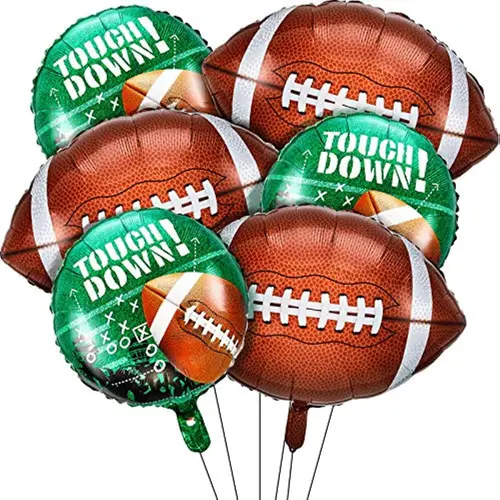This product photo showcases a bouquet of six football-themed Mylar balloons with a transparent background. The bouquet includes three large Mylar balloons shaped like footballs, complete with detailed white stitching and lines. The other three are round, green Mylar balloons featuring a football graphic over a field design adorned with X's and O's, depicting a football play, and the word "TOUCHDOWN!" in large white letters with an exclamation point. Strings hang from each balloon, giving the bouquet a cohesive look. This detailed collection highlights the vibrant and thematic football elements, perfect for sports celebrations.